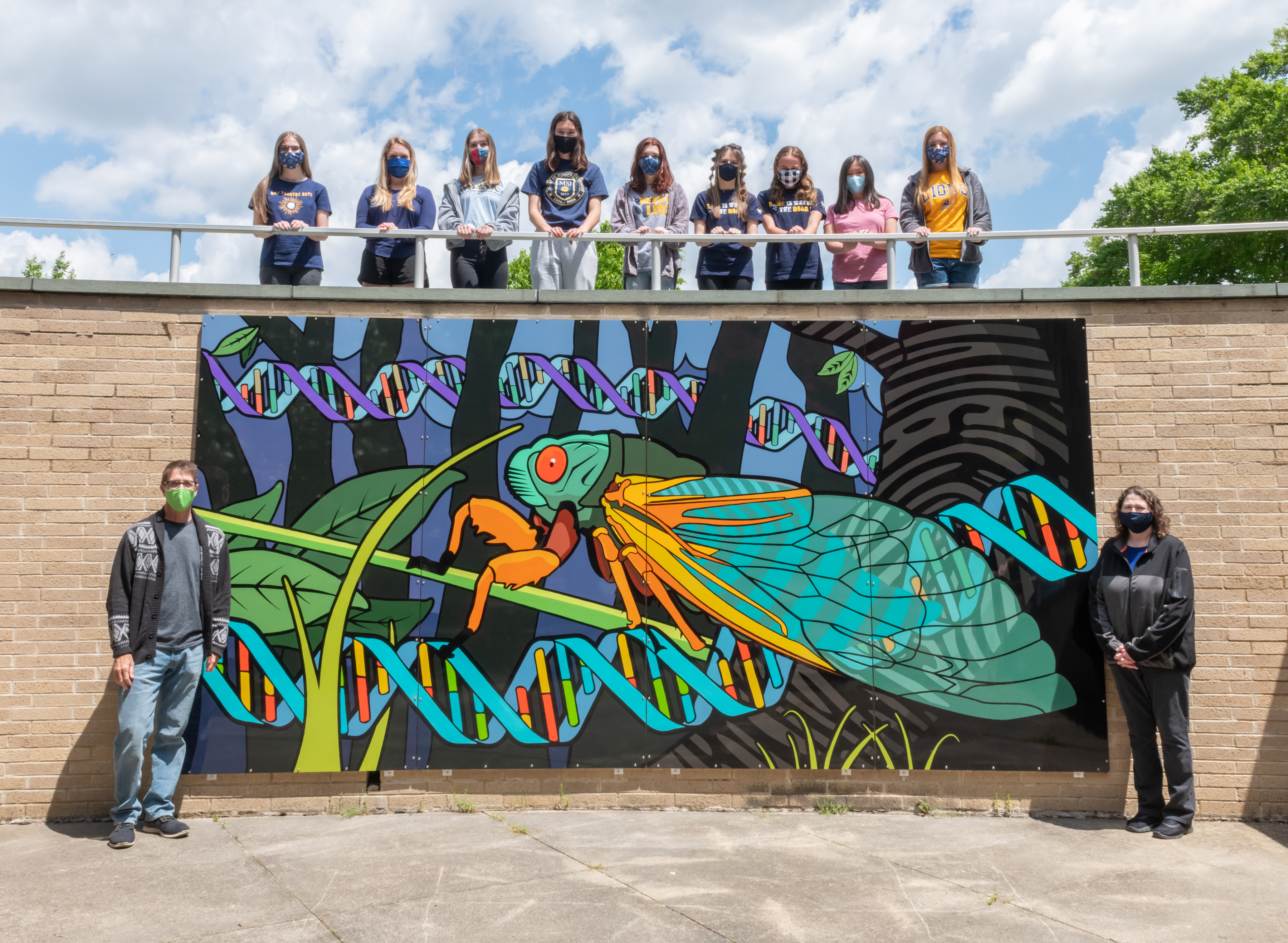This photograph captures a dynamic scene outside in front of a tall, pale brick wall, surmounted by a silver metal railing. Below the wall is a concrete slab floor where two individuals stand on either side of a vibrant mural. To the left, a man in blue jeans, a white t-shirt, and a black jacket with gray designs stands, distinguished by his bright green face mask and black-rimmed glasses. On the right, a woman in black jeans, black shoes, a gray and black jacket over a blue shirt, and a black face mask poses beside the mural. The mural itself is an intricate, cartoon-style depiction of a cricket with large blue wings, orange legs, and a red eye perched on a lime green stem, surrounded by green leaves, a dark tree featuring a gray fingerprint design, and DNA strands encircling the insect.

Above this vibrant display, nine young individuals, appearing to be students, stand behind the metal railing, gazing down at the mural. They all wear face masks and mostly don dark blue shirts, contributing to a unified appearance. This scene suggests a collaboration, likely a school club or project, highlighted by the contrast of the colorful mural against the brick and the focused, attentive posture of the students overlooking it.